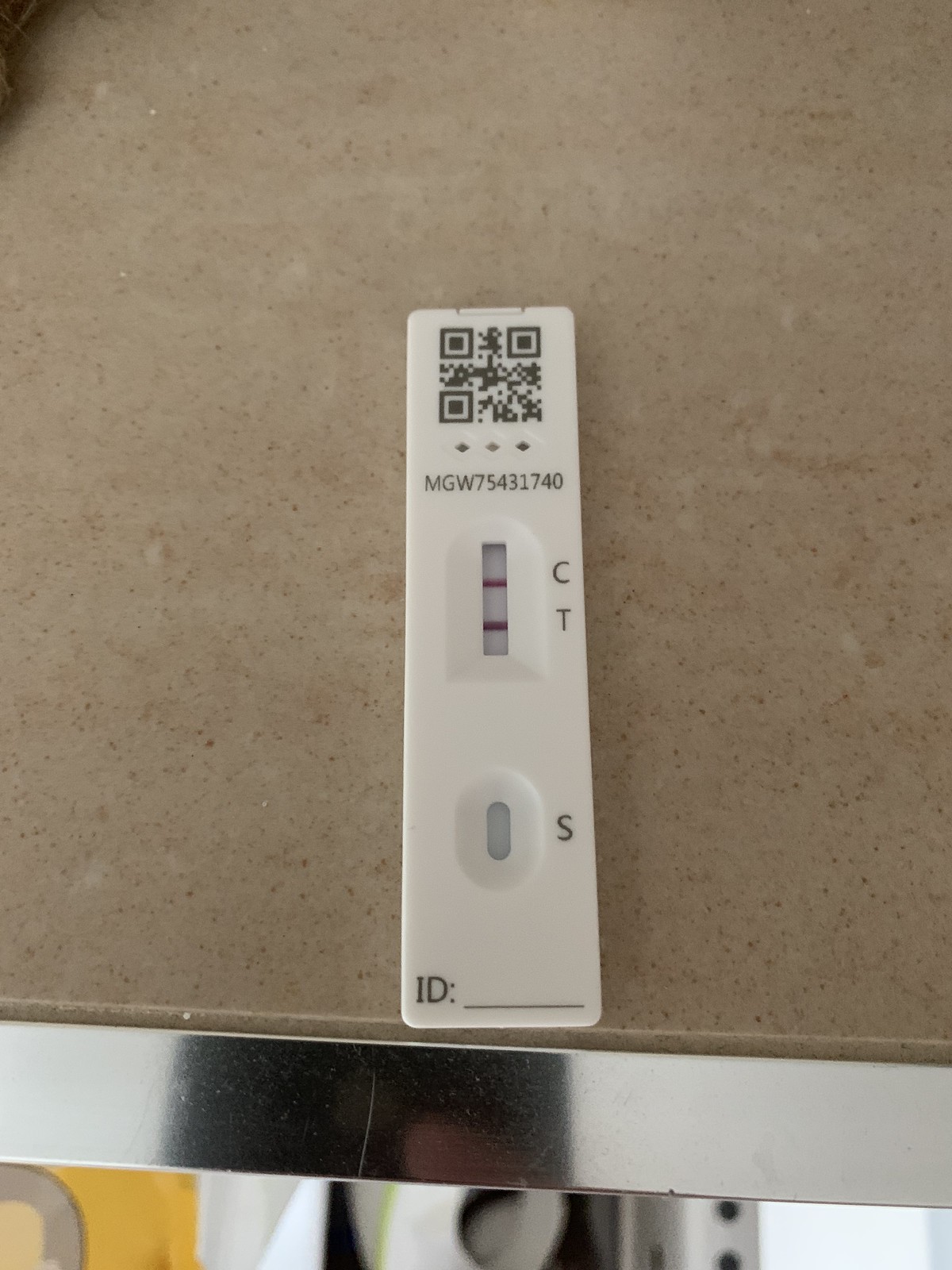The image is a top-down view of a rectangular white test strip, which appears to be either a pregnancy test or a COVID-19 test, placed on a beige granite countertop with a stainless steel trim. At the top of the test strip is a QR code, and directly below it is a model number, "MGW75431740." Midway down the test strip, the letters "C" and "T" are visible side-by-side, both marked with one red line each. Near the bottom right is the letter "S" with no markings or lines in its open slot. At the very bottom of the test strip is the designation "ID," followed by an empty space intended for an identifier. A faint reflection, likely of a cell phone being held overhead, can be seen in the stainless steel trim of the countertop.